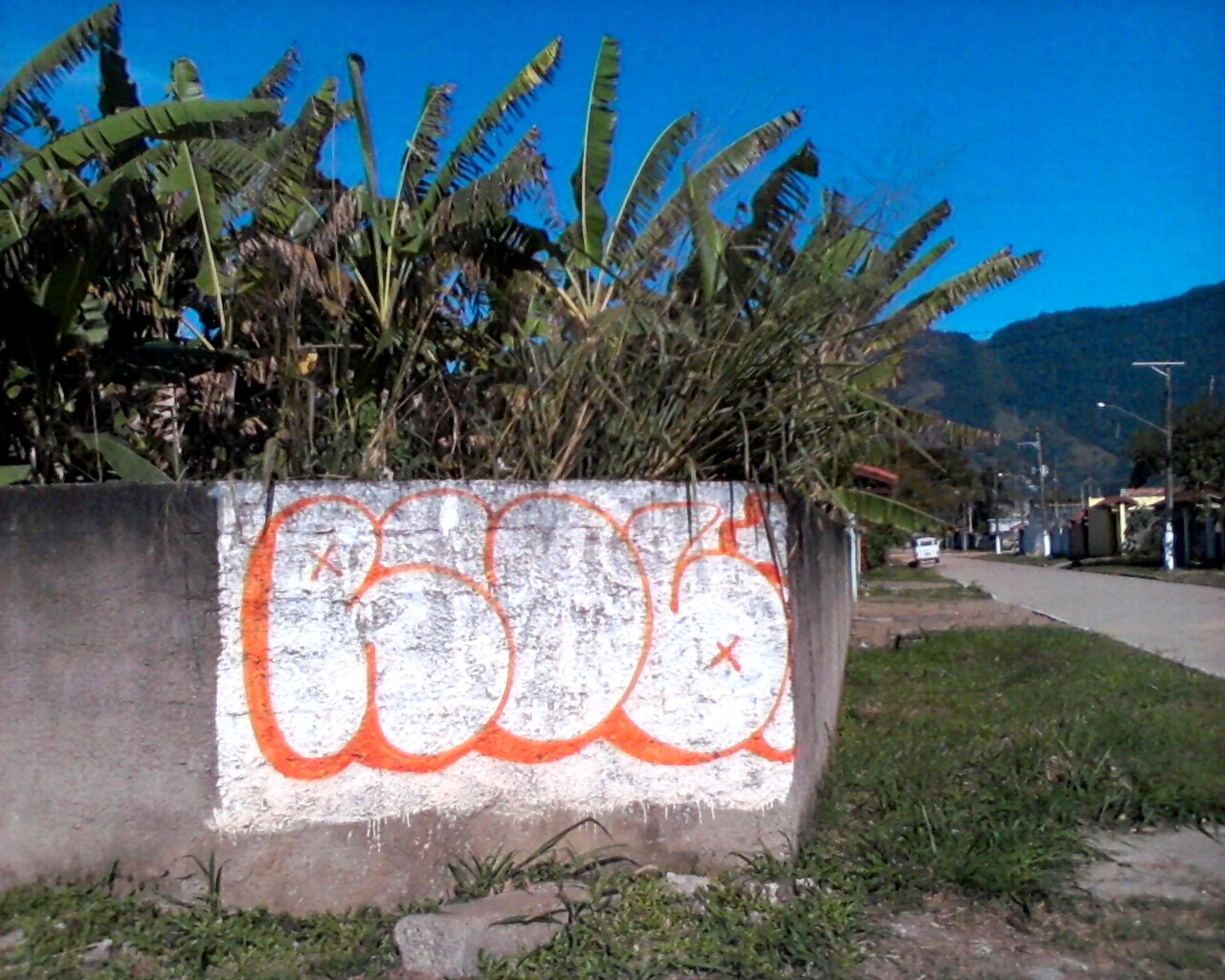This is a color photograph taken outdoors during the day, showcasing a vibrant, crystal blue sky. The central feature is a gray, weathered concrete wall that appears dirty and old, with black spots along the top edge. A prominent white rectangle with splotchy white paint and orange-outlined graffiti, comprising various roundish and egg-shaped objects with small X's, is visible on the wall. To the left of the wall is a lush row of deep green palm trees, with additional weedy branches peeking over from behind. The wall extends horizontally and then turns vertically, bordering a narrow, gray street on the right side of the image. A white vehicle is seen approaching from the distance on this street, which is lined with green grass patches and silver lampposts. The scene includes yellow and blue buildings with brown roofs in the background, and a mountainous hillside covered in green foliage on the far right.